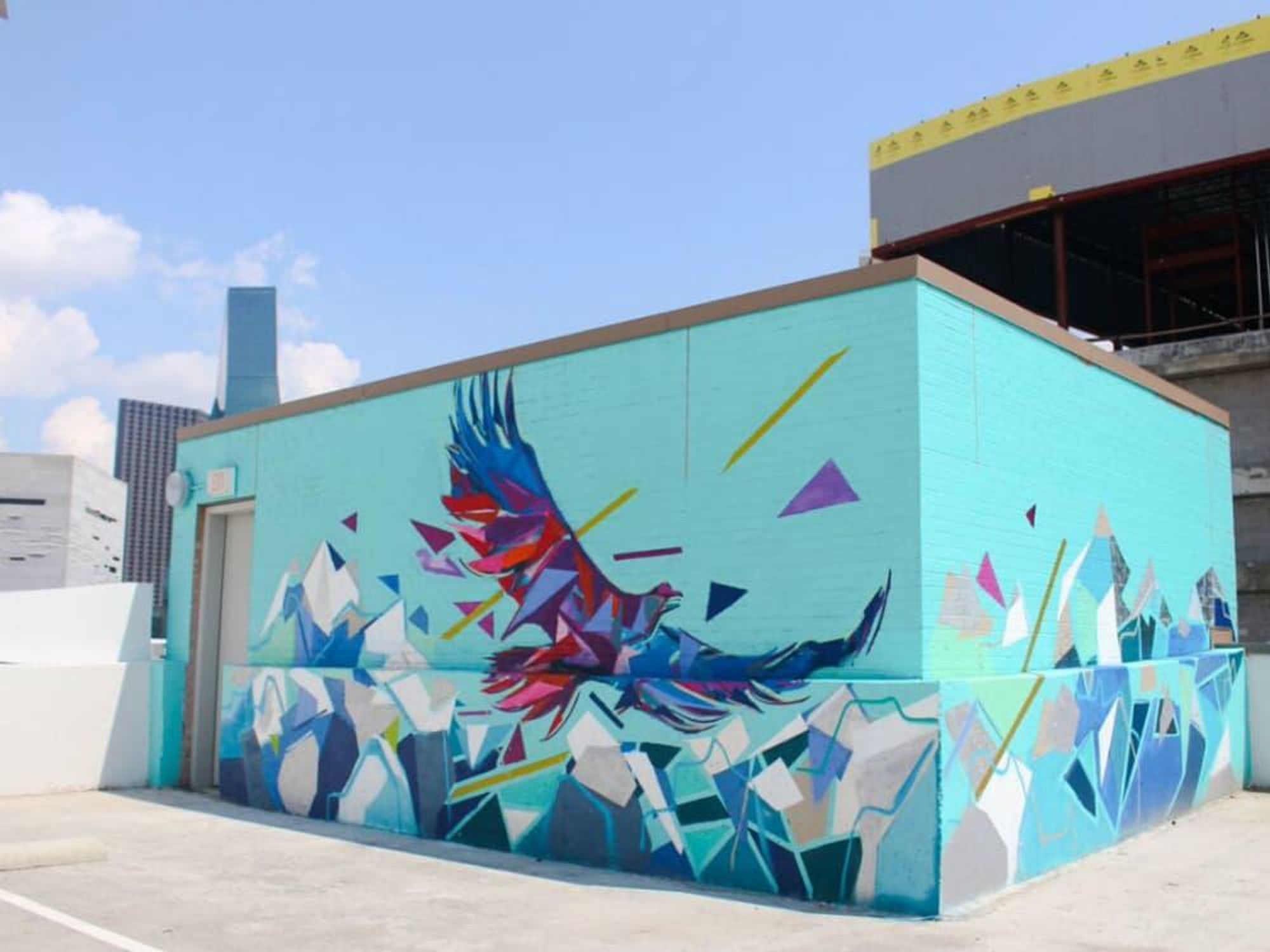This photo captures the corner of a rooftop parking lot on a smaller building, adjacent to a taller skyscraper with a yellow top and gray sides. The building on the parking lot rooftop features a detailed mural. The mural depicts a vibrant bird with dark blue wings accented with red feathers, soaring against a light blue background with geometric triangles floating around. The bottom of the mural illustrates a triangular, shard-like mountain range with white mountaintops transitioning into dark rock. The building has a gray door on its left side, serving as an entrance from the parking lot roof. Additional details in the picture include a barrier marking the parking area, a white line demarcating parking spaces, and gray asphalt beneath. The sky above is a clear blue with scattered white clouds, and a sunlit scene. In the distance, more buildings can be seen along with the scattered clouds on the left side of the image.